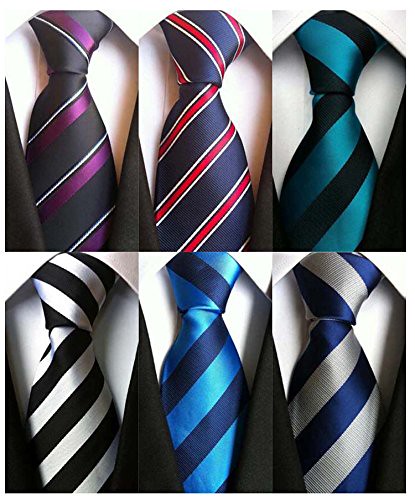This image showcases six different ties displayed against crisp white shirts and black suit coats. Each tie is adorned with diagonal stripes in a combination of unique colors. The top row features three images: The first tie is black with purple diagonal stripes, the second is blue with red and white stripes, and the third is black with turquoise stripes. The bottom row also features three ties: The first is white with black stripes, the second is a very light blue with purple stripes, and the third is purple with white stripes. All the images are evenly spaced with a bright, clear lighting that highlights the intricate designs of the ties. The ties give an impression of being worn with formal attire, possibly tucked into the suit, although it's not clearly visible whether they're on mannequins or simply arranged layouts.